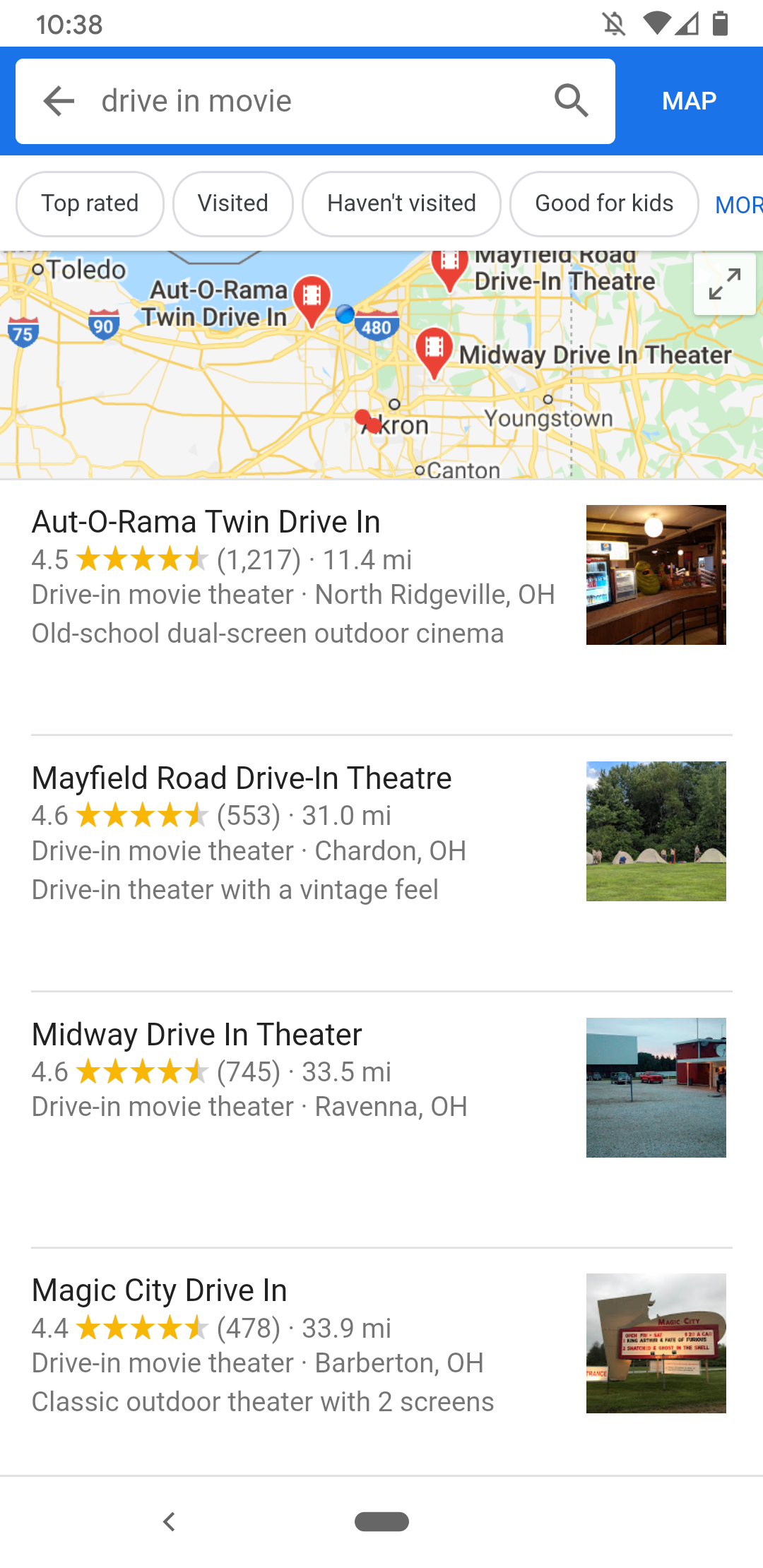The screenshot displays a search for drive-in theaters in Ohio. At the top of the screen, there is an icon with an "R" followed by the word "drive-in," alongside the current time, 10:38 PM. Various filters such as "Map," "Top Rated," "Visited," "Haven't Visited," and "Good for Kids" are also visible. 

Below these filters, several drive-in theaters are listed. The Autorama Twin Drive-In is highlighted first, boasting 12,000 reviews and located in Northridge, Ohio. It is described as an old school, dual-screen outdoor cinema.

Next on the list is the Mayfield Road Drive-In Theater in Chardon, Ohio, with 553 reviews and a rating of 4.6 stars. This drive-in is noted for its vintage feel.

The list also includes the Midway Drive-In Theater, which shares the same rating of 4.6 stars.

Finally, the Magic City Drive-In is mentioned, featuring a rating of 4.4 stars and noted for having multiple outdoor screens.